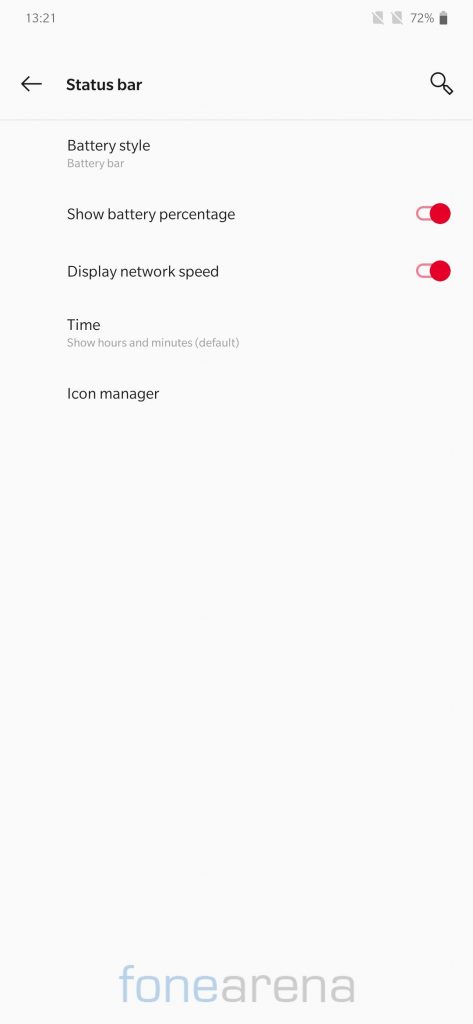This screenshot, likely taken from a mobile device, displays a settings interface on a white background. In the top-left corner, the time is shown as "13:21" in black text, and the battery level is next to it at 72%. Below, on the left-hand side, there's a left-facing arrow and the word "Status bar" in bold black text. On the far right, there's a magnifying glass icon for search functionality.

A faint gray line separates this header from the main settings options below. The first option listed is "Battery style" in black text, with "Battery bar" in gray text beneath it. The next line features "Show battery percentage," accompanied by a slider that is red and toggled to the right, indicating that this option is enabled.

The third line down is "Display network speed," again accompanied by a red slider toggled to the right. The fourth option, "Time," has a sub-option "Show hours and minutes (default)" written in light gray below it.

The last item on the list is "Icon manager," also in black text. At the very bottom of the interface, "PhoneArena" is displayed, with "Phone" in blue and "Arena" in gray text, implying the source or application name.

Overall, this screenshot illustrates a status bar settings menu where users can customize various aspects such as battery style, network speed display, and time format.